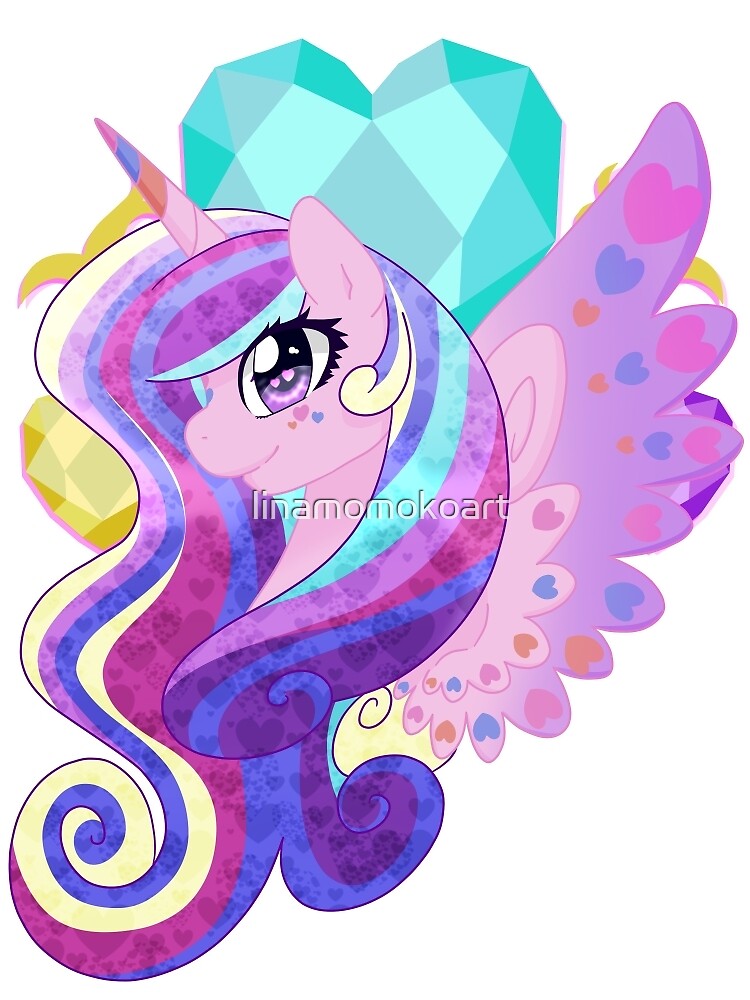This image is a captivating digital art piece featuring a My Little Pony-inspired unicorn with an exquisitely detailed and colorful appearance. The unicorn's body is light pink, adorned with extraordinarily long, wavy hair that cascades down her neck in a vibrant combination of purple, pink, blue, turquoise, and yellow. Her enormous, anime-inspired eyes, complete with long lashes, have irises colored in shades of purple. Cute, heart-shaped freckles embellish one side of her face, adding a whimsical touch.

Protruding from her head, the unicorn's horn is swirled with shades of pink, orange, and blue. Positioned at a three-quarter angle to the left, she displays one sizable, elaborate wing decorated with multicolored hearts along the feather edges. The inside of the wing is predominantly light pink, transitioning into hues of purple and additional pink tones. 

Behind the unicorn, a large turquoise heart, faceted like a gemstone, serves as a striking backdrop, alongside a smaller yellow faceted gem heart. Additional decorative yellow swirls, possibly filigree, add to the overall enchanting design. A watermark reading "Lina Momo Co-Art" is present across the center of the image, marking the artist's signature. This fantastical depiction seamlessly blends modern cartoon aesthetics with intricate, colorful details that make the composition truly stand out.